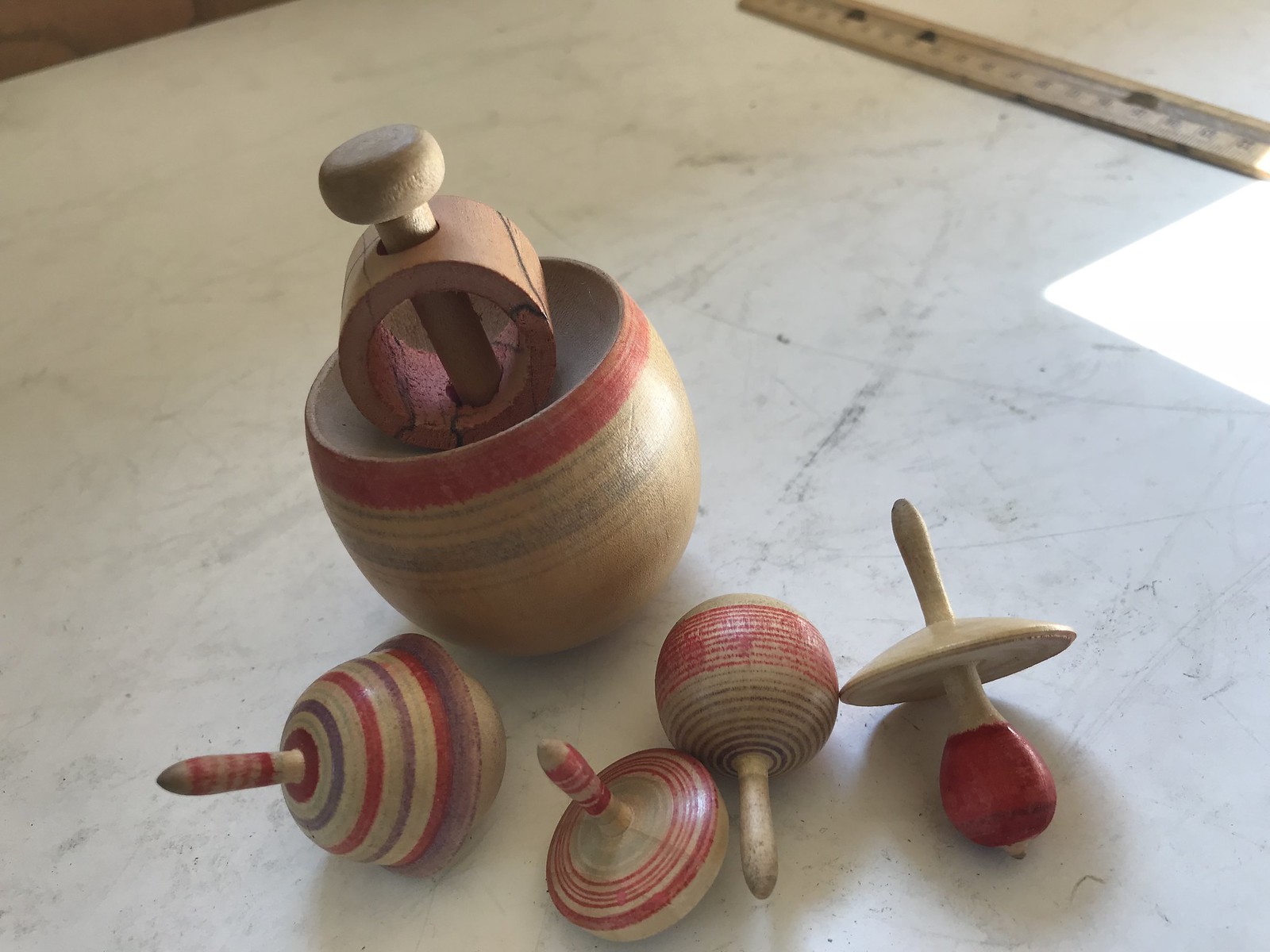The image depicts a selection of wooden spinning toys arranged on a white granite surface, which has noticeable scratches and marks. In the background, a 12-inch wooden ruler lies diagonally in the top right corner along with a piece of white paper partially visible. The forefront features five intricately designed, circular wooden toys. The largest toy resembles a pot with a distinctive handle, adorned with red and green lines. Another smaller toy, situated at the bottom left, has a dreidel-like shape, sporting red and purple lines and a small handle at the end. Among the other pieces, there's one resembling a maraca and another that looks like a pacifier with a red tip. All the toys share a common light brown wood color with vibrant red and other colored designs.